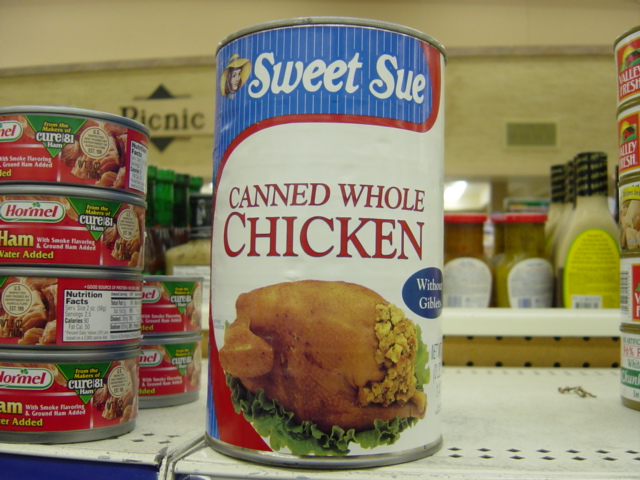The image depicts a notable can of Sweet Sue Canned Whole Chicken prominently placed on a shelf in a grocery store. This can, primarily white with red accents and blue detailing, features a label with the text "Sweet Sue" at the top along with an image of a woman. The bulk of the label displays an appetizing roast chicken, complete with stuffing, resting on a bed of rough lettuce leaves. A blue lozenge also clearly states, "Without giblets." The can is flanked by other items: to the left, a stack of six small Hormel canned ham tins with red labels, and to the right are five slender, unidentified cans. In the background, bottles of salad dressing are visible on an opposite shelf, along with an out-of-focus sign reading "Picnic" featuring triangular arrows above and below it, implying this section might pertain to picnic-related goods. The can of Sweet Sue Canned Whole Chicken is unmistakably the central feature of this image, standing out against its grocery store surroundings.